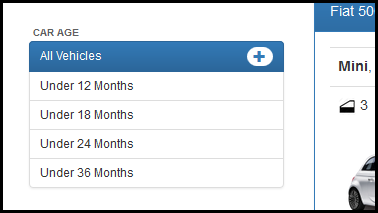The image features a white background bordered on all four sides by a black border. In the top right corner, there is a small dark blue rectangle with the number "550" written in white text. Below this, along the left side of the image, runs a vertical light blue line extending from the top to the bottom.

To the right of this line, the word "MINI" is displayed in bold black text. Adjacent to the word "MINI" is a logo which is half white on the top and black on the bottom, accompanied by the number "3" beside it. Below this logo, a partial white car is visible, showing only the very rear of the vehicle.

On the left side of the image, near the top in gray capital letters, appears the text "CAR AGE." Underneath "CAR AGE," a blue rectangle with white text reads "ALL VEHICLES." To the right of this blue rectangle is a circle containing a blue plus symbol.

Below this section are several subsequent boxes, each with a white background. The first box is labeled "UNDER 12 MONTHS," followed by another box labeled "UNDER 18 MONTHS." Below these, there is a third box labeled "UNDER 24 MONTHS," and at the very bottom, a fourth box labeled "UNDER 36 MONTHS."